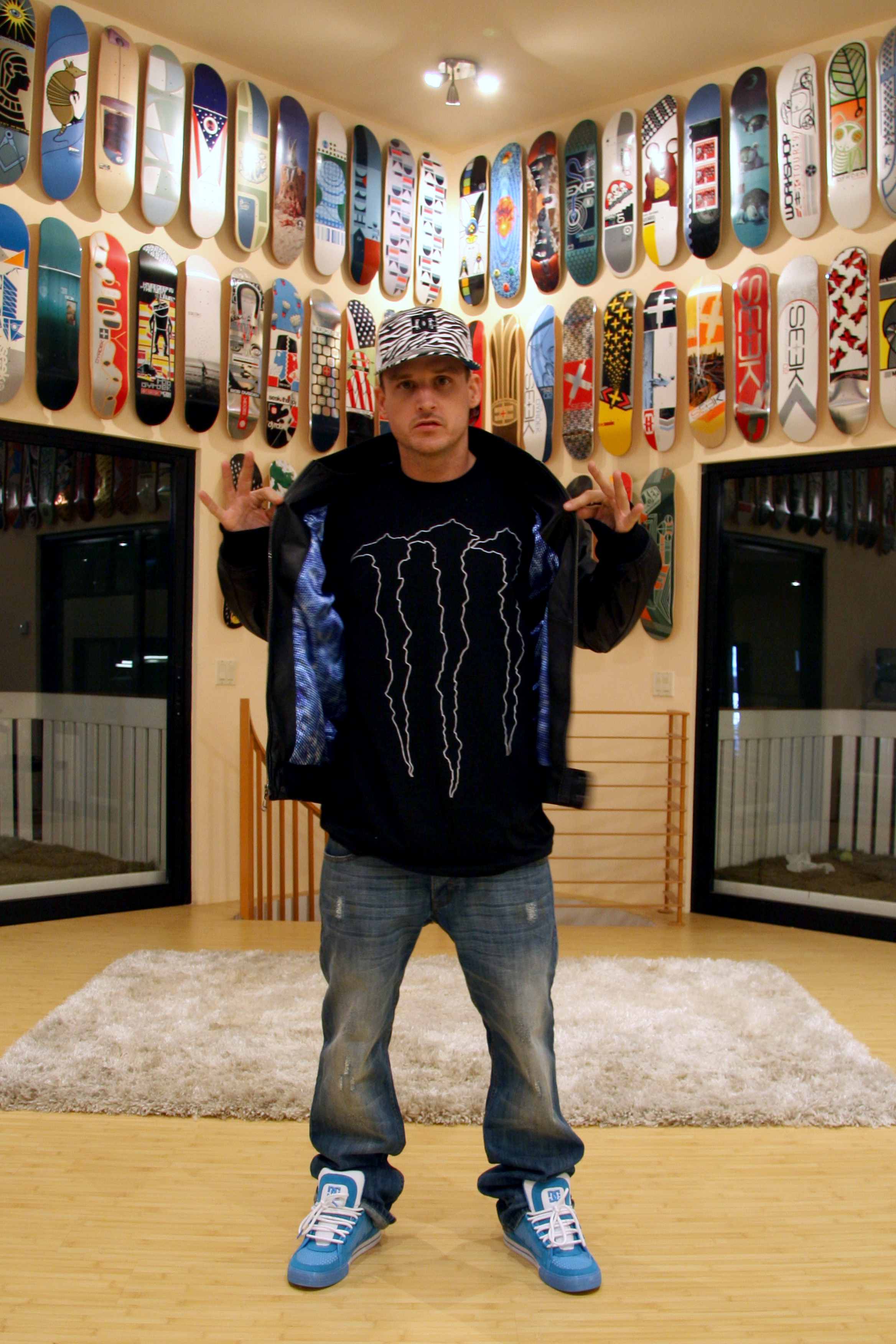This is a detailed color photograph of a young Caucasian man in his 20s or 30s standing in the center of an expansive room with carefully arranged skateboards or electric skateboards hung on the walls. The room features a light-colored wooden floor with a small rectangular shaggy rug beneath the man. Behind him is a curved metal staircase descending to a lower level. The walls and ceiling are painted a tan-gray color and adorned with approximately 30 skateboards in various designs, meticulously lined up in two rows. Adjacent to him on either side, the room has two large rectangular windows that reveal a nighttime scene outside.

The man is dressed in a black jacket with teal blue lining, an intricate black T-shirt featuring three long, pointed claw-like symbols, faded blue jeans, and aqua blue sneakers. He also sports a black-and-white patterned baseball cap. He stands facing the camera with his hands raised, pinching his thumb and second finger together in a gesture. His facial features include small inset eyes, prominent ears, a definitive nose, and a shadow of mustache and beard. The overall ambiance of the photograph is subtly illuminated by a three-bulb light fixture on the ceiling, contributing to the warm and inviting aesthetic of the room.